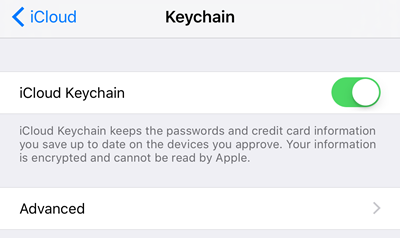The image is a screenshot of an iPhone's settings, specifically highlighting the iCloud Keychain feature. At the top, there is the word "iCloud" followed by "Keychain" in larger text. Below this, there is a green toggle switch indicating that Keychain is enabled. 

Beneath the toggle, there is a detailed description inside a gray rectangle, explaining the function of iCloud Keychain: "iCloud Keychain keeps the passwords and credit card information you save up to date on the devices you approve. Your information is encrypted and cannot be read by Apple."

Additionally, there is a partial text reading "iAns" visible at the bottom, signifying possibly a cropped or partially obscured section of the screen. The overall color scheme of the image is predominantly gray, with splashes of white here and there. The top left of the screen also features blue text. This detailed depiction captures the interface and critical information of the iCloud Keychain settings on the user’s phone.